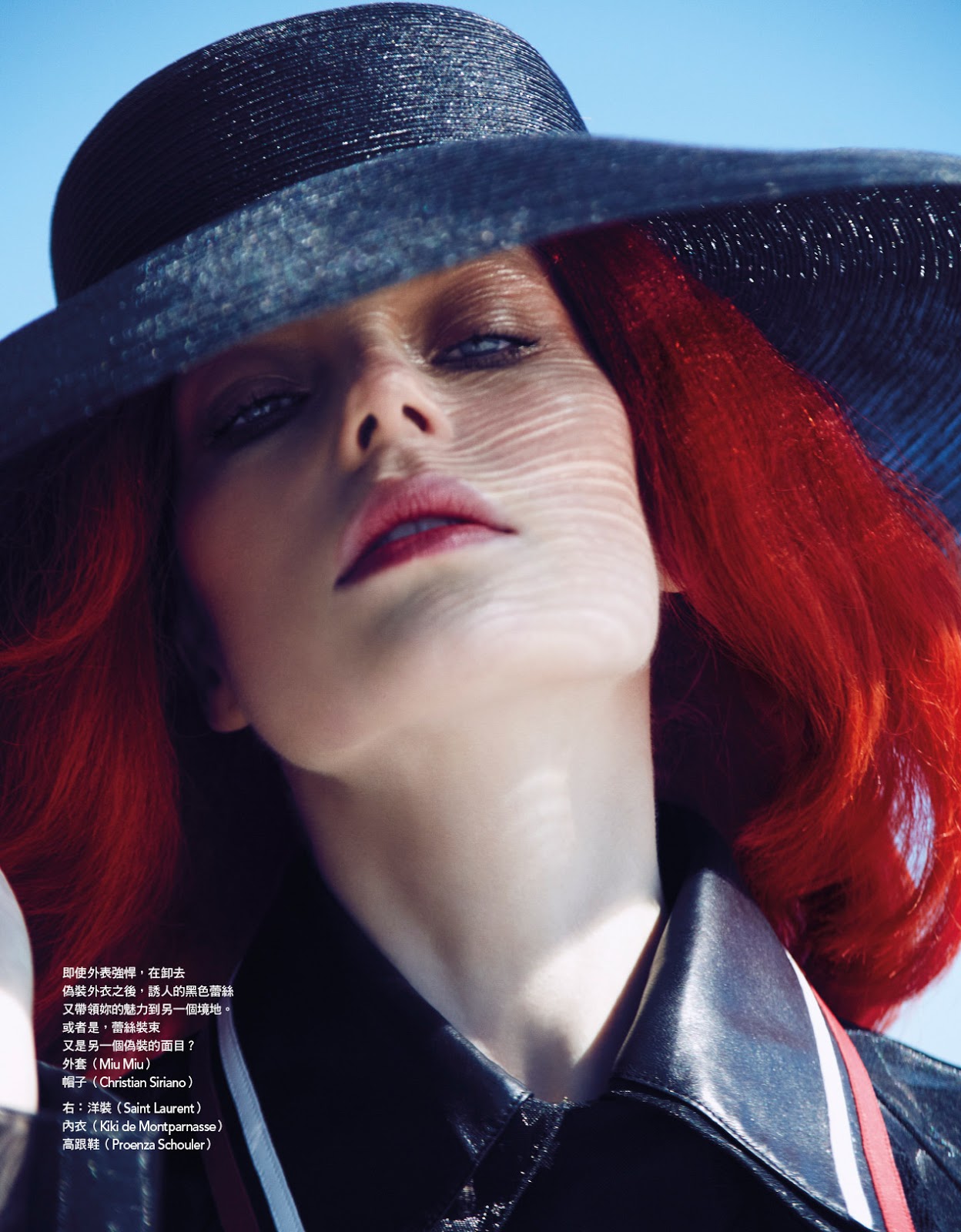The image features a close-up of a woman with dyed, vibrant red hair, shaded slightly orange, cascading to her shoulders. She dons a black straw sun hat, casting intricate shadows across her fair, pale face, suggesting she’s outdoors. Her blue eyes, enhanced with brown eyeshadow, gaze directly at the viewer with a smoldering, intense look, giving the picture a sophisticated, model-like quality. Her slightly parted lips are tinted a subtle red. She is dressed in a black, leather-like collared top, accented with white and red stripes. At the bottom left corner of the image, there is small text, possibly in Chinese, Japanese, or Korean, listing high-end fashion names like Miu Miu, Christian Siriano, Saint Laurent, Kiki de Montparnasse, and Proenza Schouler, indicating the brands she might be wearing. The background shows a small sliver of blue, reinforcing the outdoor setting, with no other objects visible. The overall expression of the woman is neutral, accentuating the stylistic and atmospheric tone of the photograph.